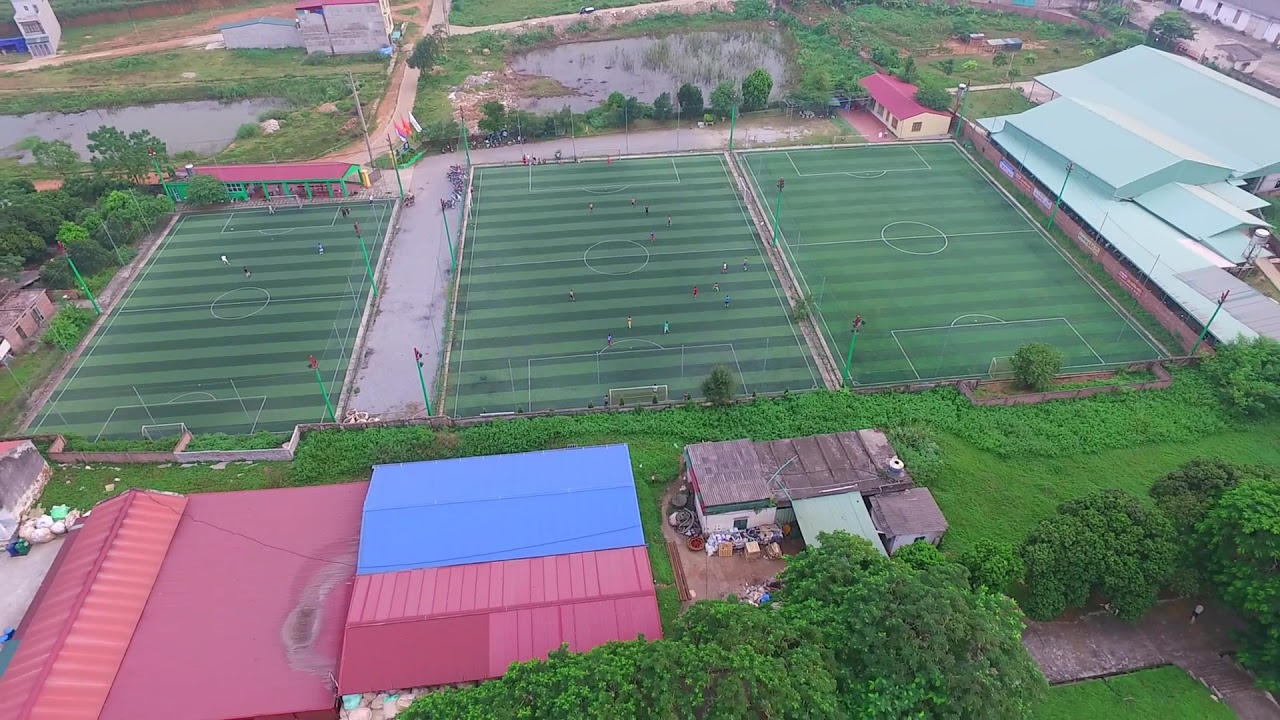This semi-aerial view captures a vibrant scene centered around three soccer fields, each meticulously mowed into alternating light and dark green stripes. The left and middle fields, particularly bustling with activity, feature players clad in assorted colors—green, blue, red, yellow, white, and black—suggesting a lively practice session rather than a formal match. Spectators surround the fields, adding to the dynamic atmosphere. In contrast, the right field appears empty.

The foreground reveals rooftops with distinctly colored tiles: pink and turquoise with a blue tarp and a light turquoise roof in the top right. Further afield, there's a mix of natural and urban elements—lush green trees and lawns, a glistening body of water in the top middle, patches of dirt, and scattered buildings. A longer white-roofed structure stands out on the right side, completing the picturesque landscape.